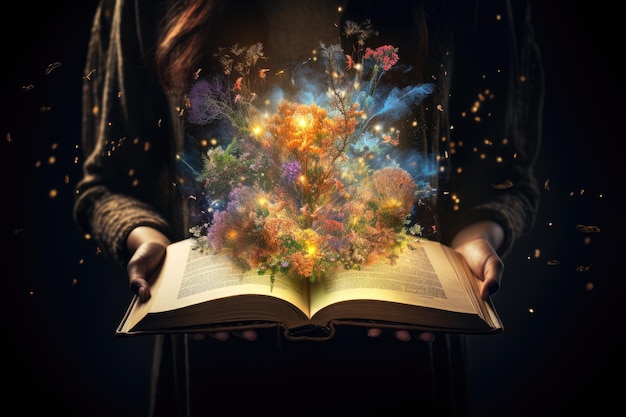The image is a captivating horizontal, rectangular artwork that blends photography with CGI enhancements, resulting in a hyper-realistic depiction. It shows a person, whose light-colored skin and long, flowing red or brunette hair hint at their appearance, holding an open book with outstretched arms. This person is dressed in a dark-colored robe or a long black coat. The main focus is the book, from which an enchanting, magical scene emerges. The book itself has gold-tinged pages adorned with black ink text on white sheets. Bursting forth from the book is an imaginative universe that resembles a vibrant, glowing garden. The garden displays a mesmerizing array of colors—blue, pink, yellow, orange, and green—with flowers that look drawn rather than real. Glowing speckles of light, reminiscent of gold confetti and glitter, float out from the book, creating an atmosphere of wonder against the stark, black background. This powerful visual metaphorically illustrates the transformative power of reading, suggesting that through books, one can escape into fantastical, otherworldly realms.